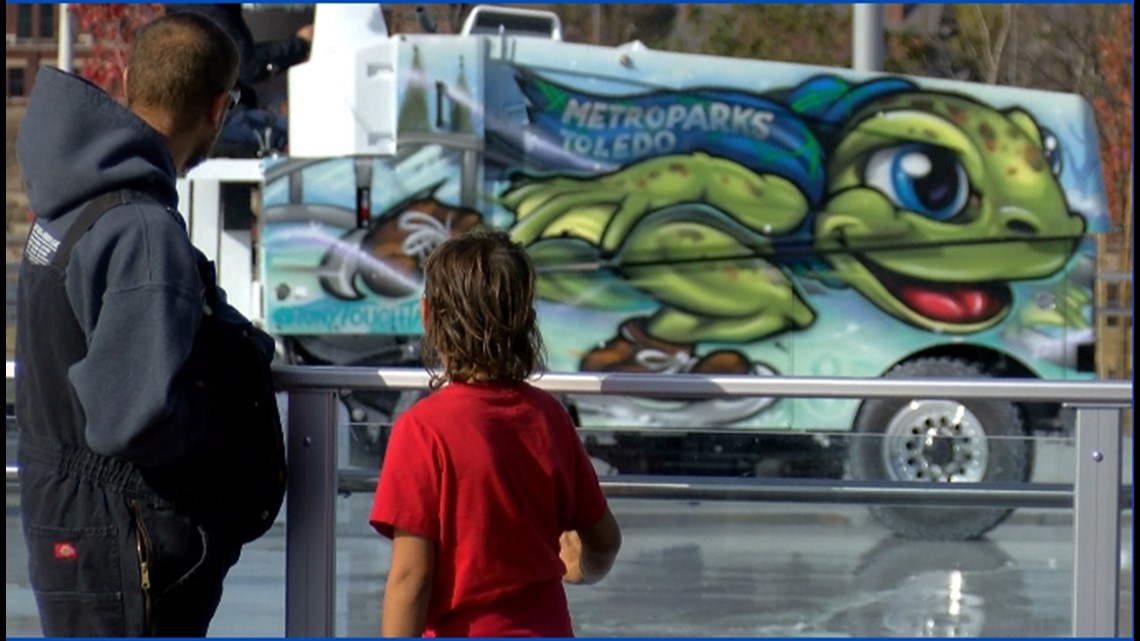In the photograph, a young boy with shoulder-length brown hair, wearing a red short-sleeved shirt, stands beside a man with close-cropped brown hair, dressed in a gray hoodie and black jeans. They are outside on a wet, reflective ground, and the sun is shining. They are standing behind a glass railing and appear to be looking at a nearby white truck. This truck has shiny wheels and features a large mural of a green frog with a caricatured large head, black pupils, and blue eyes. The frog, dressed in a blue beanie and a scarf that reads "Metro Parks Toledo," is depicted ice skating against a light blue background. Surrounding the scene are trees with fall foliage.